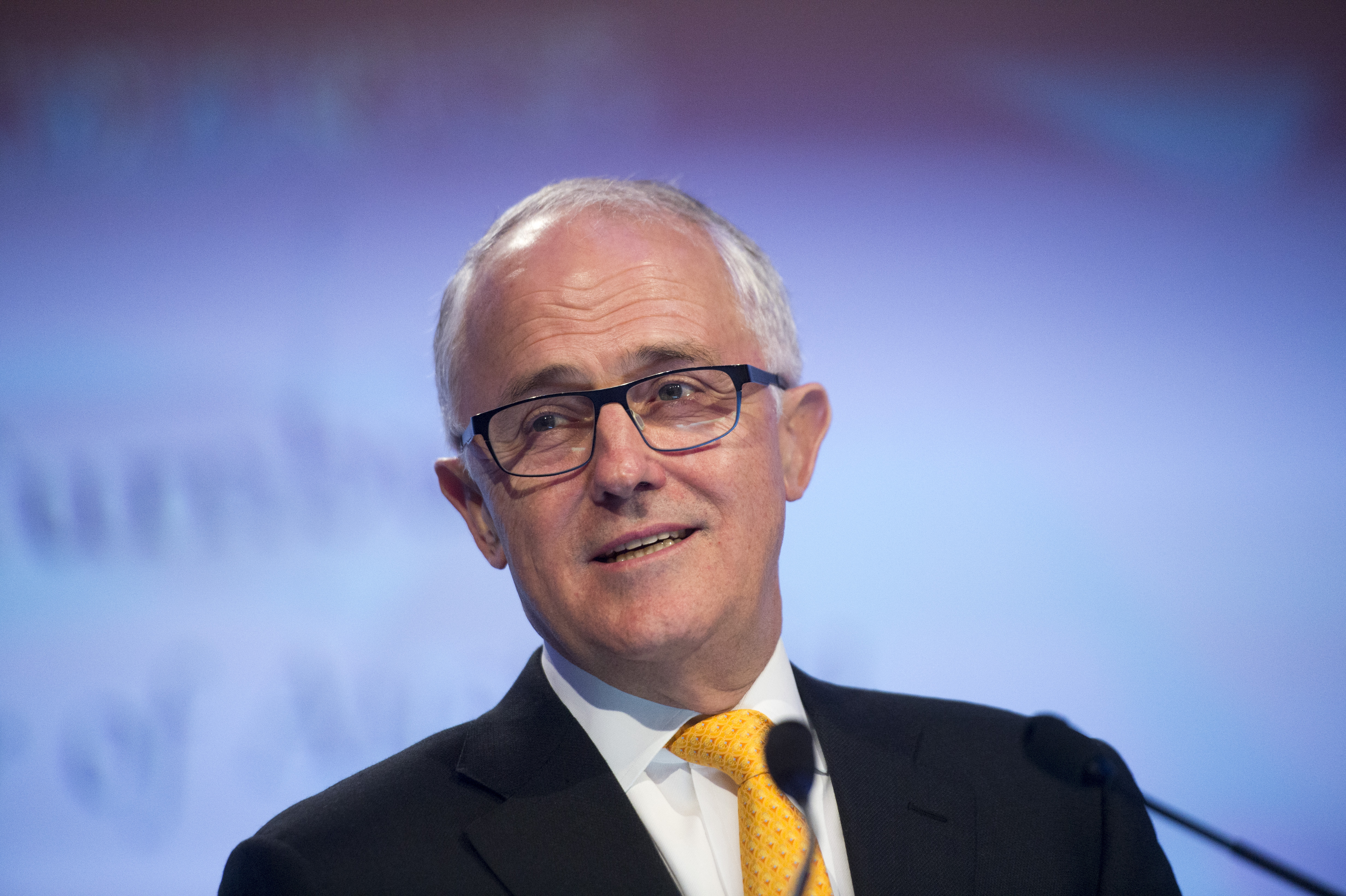In the photograph, there is a Caucasian man with a balding head and silver hair on the sides, wearing black-framed eyeglasses and a white button-down collared shirt. He sports a bright orangish-yellowish, gold-colored tie paired with a dark blue suit jacket. The man's head and upper torso are visible, and he appears to be tilted slightly to the left, with his mouth open, showing both rows of teeth, suggesting he is speaking. In front of him are two slightly out-of-focus black microphones positioned at the lower middle and lower right. The background features a gradient transitioning from white in the center to blue and then black towards the edges, with indistinct black text in the middle.